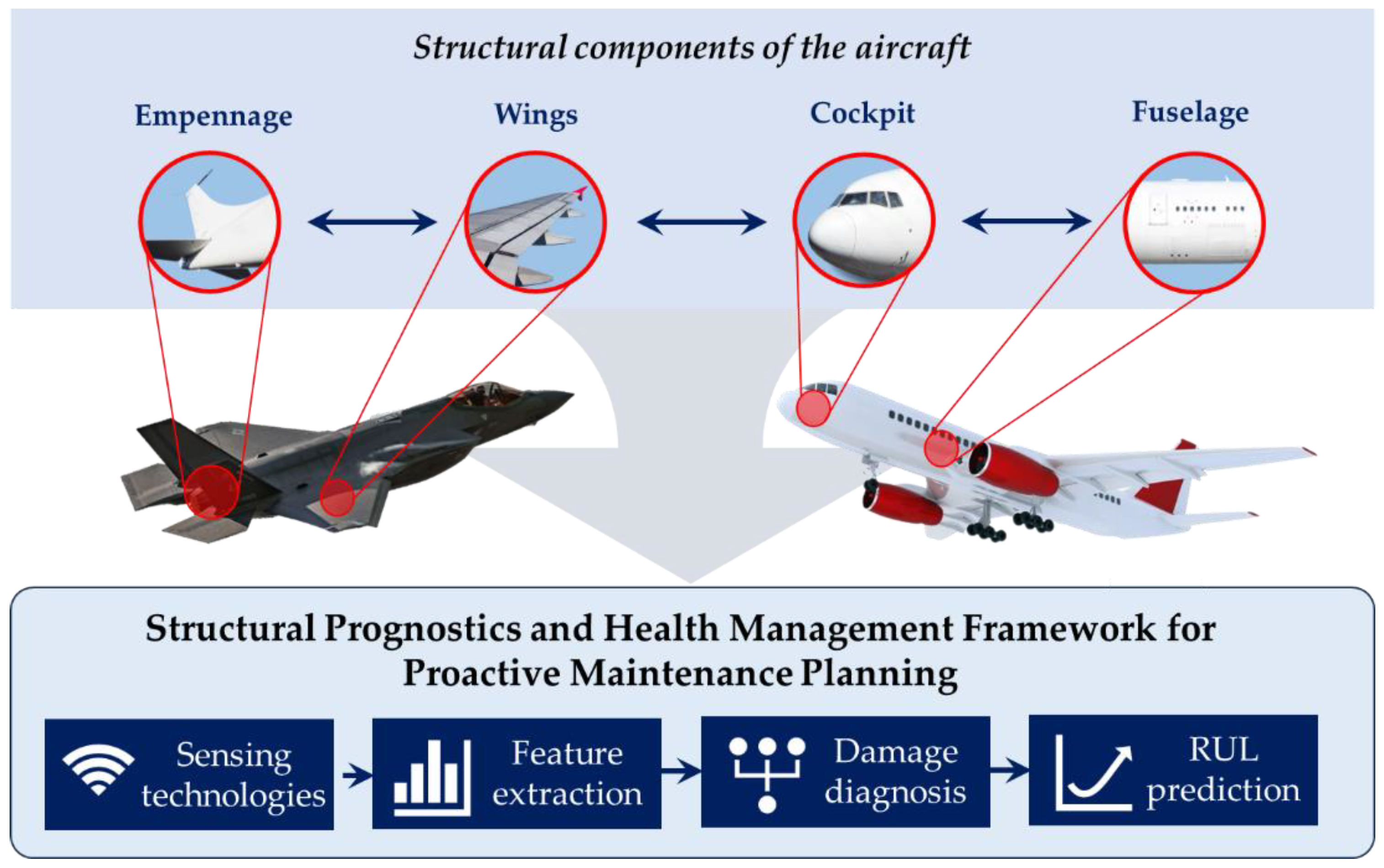The image depicts a detailed diagram titled "Structural Components of the Aircraft," which outlines the key structural parts of two different types of aircraft: a military jet, in gray-black, and a commercial passenger plane, which is white with red engines and a red tail. The diagram highlights essential components of both aircraft, including the empennage (tail), wings, cockpit, and fuselage, with circles around each part for emphasis. Beneath this, a rectangular horizontal box reads "Structural Prognostics and Health Management Framework for Proactive Maintenance Planning," followed by four blue-background rectangles labeled as "Sensing Technologies," "Feature Extraction," "Damage Diagnosis," and "RUL Prediction," with arrows directing the flow between these components. The overall aesthetic includes a blue section at the top which introduces the structural components, and the layout is divided into descriptive segments with both visual and textual elements to facilitate understanding of the aircraft's maintenance planning framework.